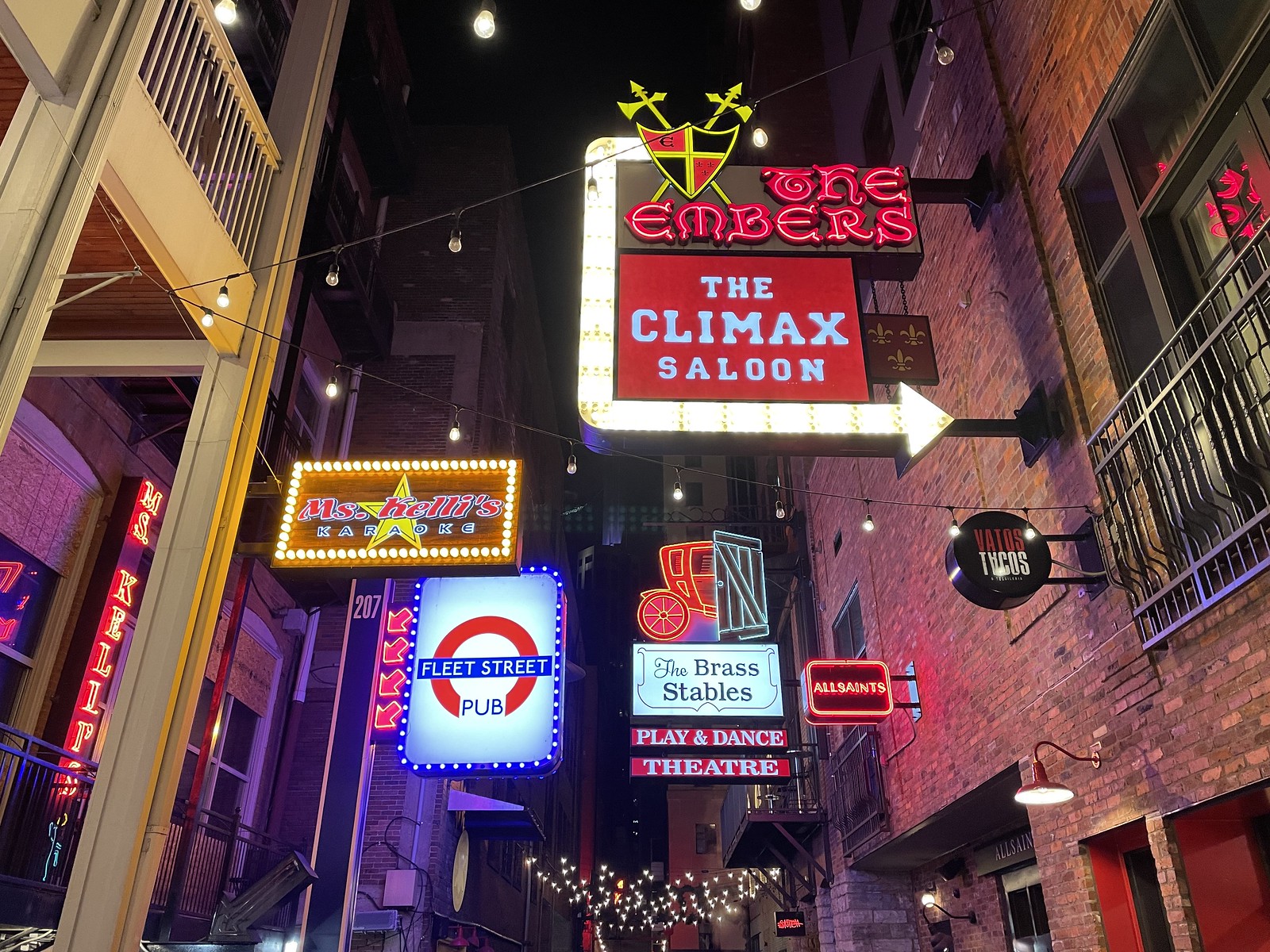The image features a bustling cityscape dominated by numerous tall buildings flanking both sides. The urban environment is characterized by its dense array of structures, devoid of any visible greenery such as trees. Prominently displayed on one of the buildings is a collection of distinct signs. 

At the forefront, a sign reads "The Embers" accompanied by a shield emblem. The shield is outlined in yellow and partitioned into four segments filled with red and black, and features two crossed axes protruding from it. Just beneath this, a vibrant red square background highlights the text "The Climax Saloon" in white, alongside a large arrow that directs towards the building.

A notable balcony with metal bars is visible, featuring windows and a door. Below this balcony, another sign spells out "Yato's" with the 'A' intriguingly presented upside down. This sign, set against a black circular backdrop with red and white text, suggests it might be a taco shop, though the small size makes it slightly difficult to decipher. 

Another sign identifies "The Brass Stables," illustrated with a wagon and a barn door. This digital sign brightly advertises the place as a "Play and Dance Theater." Surrounding signs further add to the urban texture, including ones for "Fleet Street Pub" and "All Saints," contributing to the city's vibrant, commercial atmosphere.